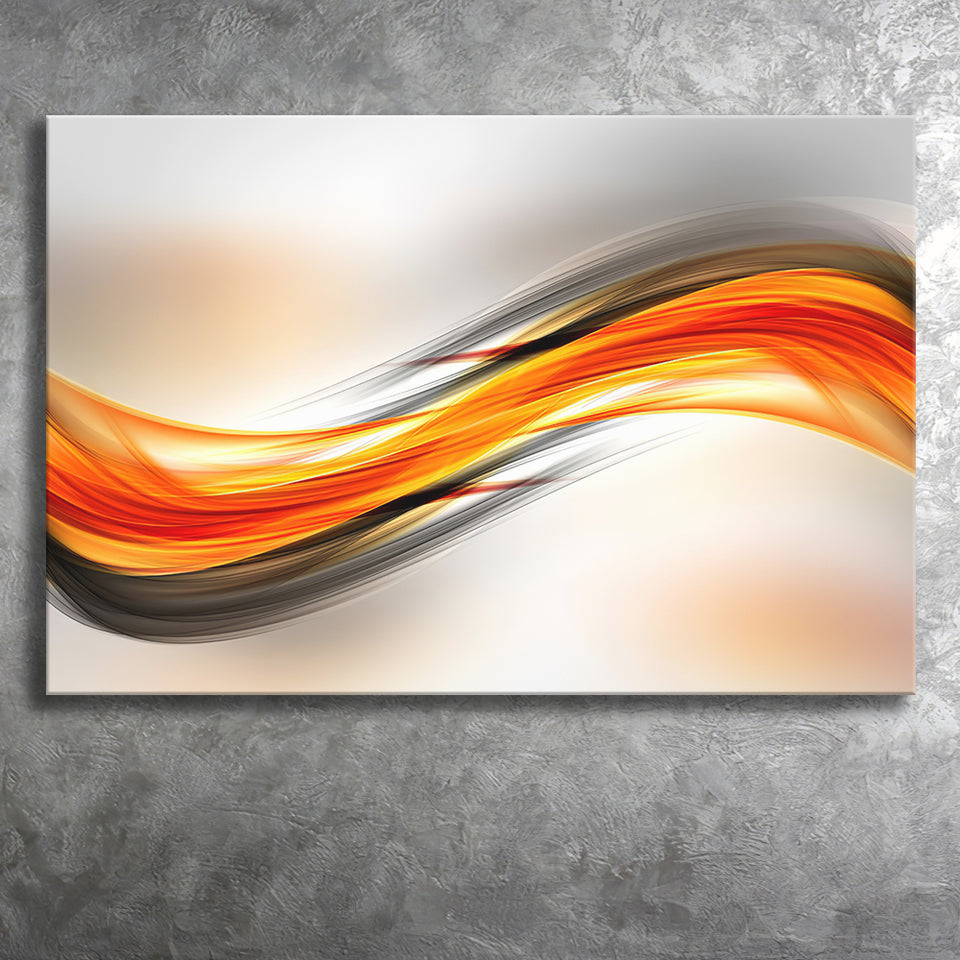The artwork displayed is on a white canvas hanging against a marbleized gray wall. The painting predominantly features a mixture of gray and varying shades of orange, including a lighter tone. The upper half of the canvas is more gray, while the lower half transitions to white with splashes of orangish hues concentrated in the lower right corner. The design consists of slight, horizontally-oriented brushstrokes that create a dynamic, swirling pattern, reminiscent of fire. Additional dark streaks, notably in shades of brown and dark gray, cut through this fiery swirl, with some lines extending fully across the canvas while others stop halfway, enhancing the overall texture and movement within the artwork.